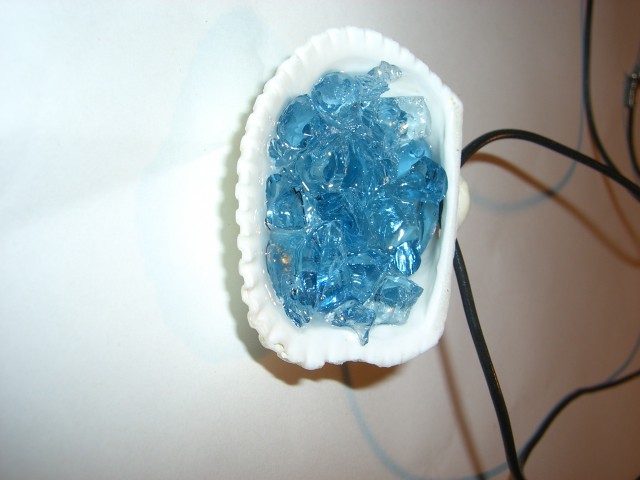This photo showcases a striking white clam shell with distinct ridges around its edges, positioned on a white background. The clam shell's interior cradles an intriguing blue crystalline material, reminiscent of a clear, light blue ocean, adding a mesmerizing, almost translucent quality. Behind the shell, black wires stretch across the white backdrop, casting intricate shadows that add depth and a subtle bluish tint to the scene. Towards the upper right, an attachment, possibly anchoring the wires to the wall, is faintly visible amidst the shadows, though its exact nature remains ambiguous. The combined elements of the clam shell, the blue crystals, and the shadowed wires create a captivating and mysterious composition.